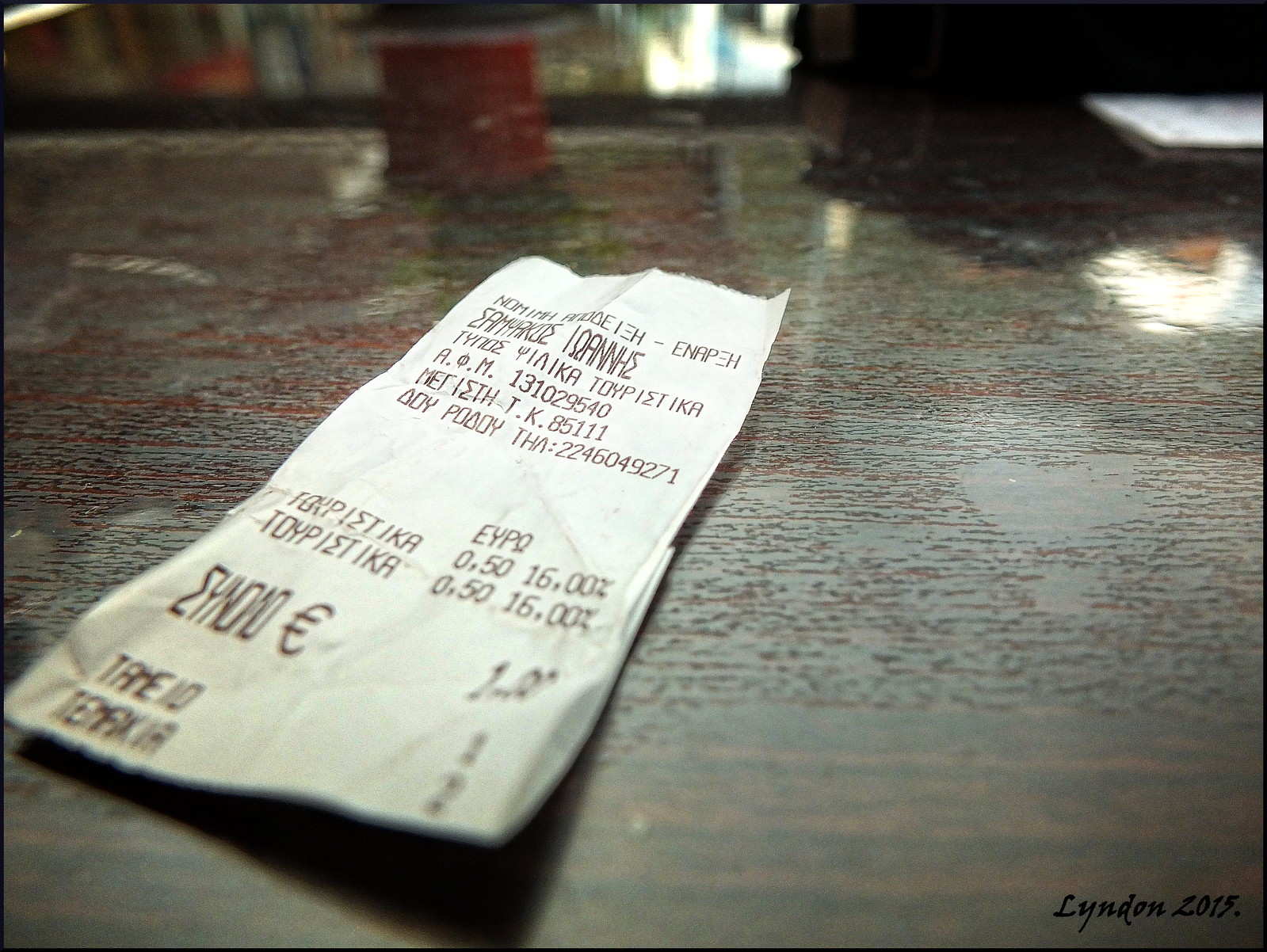A close-up image of a white, crumpled receipt, written in what appears to be a foreign language, likely Russian, lies at an angle on a highly reflective, lacquered wooden table that has a grayish or dark brown hue. The table's polished surface mirrors some objects, faint daylight, and a red item, suggesting a possible bar counter or similar setting. The receipt, partially folded, displays numbers and text that don't clearly reveal a total price but mention an item quantity of 1.00. Blurry light can also be seen in the upper middle background of the image. On the bottom right corner of the receipt, "Linden 2015." is printed.